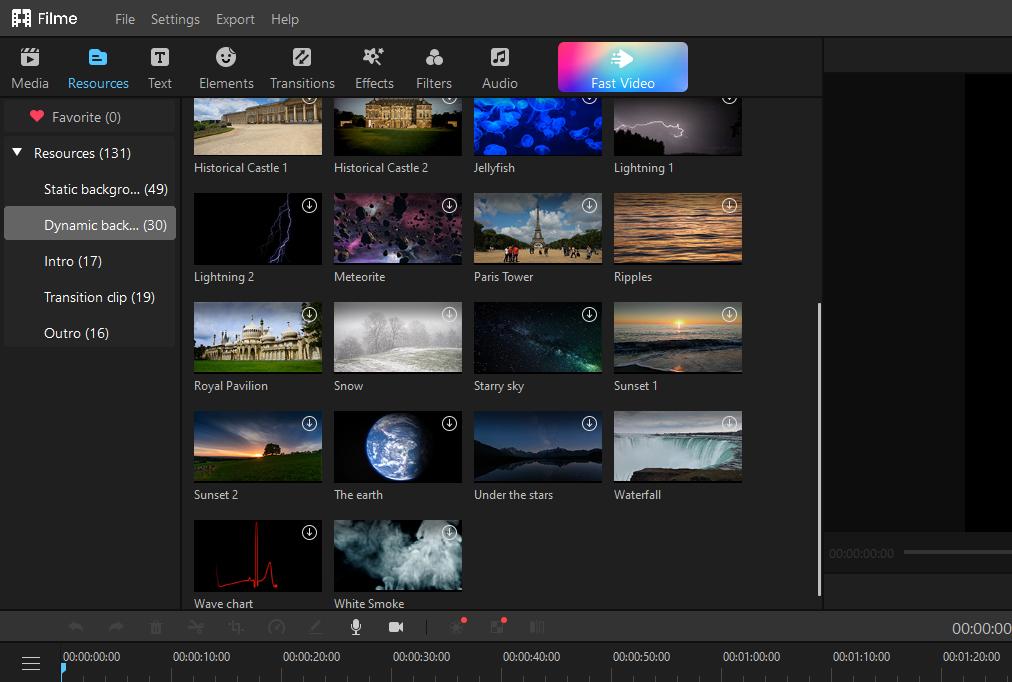This image is a screen capture of video editing software, displaying its interface and available resources. 

At the top of the interface, the menu bar is positioned against a black background with a mix of gray and white text. It prominently features the title "Filme," accompanied by a white film strip icon. The menu includes options such as "File," "Settings," "Export," and "Help."

Below the menu bar, a series of gray icons represent different tools within the software:
- "Media" with a clapboard icon featuring a play button.
- "Resources" marked with a blue folder icon.
- "Text" with a "T" enclosed in a square.
- "Elements" symbolized by a smiling emoji face.
- "Transitions" denoted by an up and down arrow.
- "Effects" illustrated with a magic wand and star.
- "Filters" represented by three interlocking circles.
- "Audio" shown with a music note inside a square.
- "Fast Video" with a play button situated in a multicolored (pink, blue, and teal) box.

A collection of labeled thumbnails dominates the middle section of the screen, each described in white font:
- "Historical Castle One" depicts a tan castle.
- "Historical Castle Two" features a stately tan castle on a grassy area.
- "Jellyfish" shows blue jellyfish.
- "Lightning" captures a lightning strike against a black sky.
- "Lightning Two" presents a lightning bolt against a navy sky.
- "Meteorite" illustrates dark gray meteorites hurtling through a vivid pink and purple space.
- "Paris Tower" displays tourists visiting the Eiffel Tower.
- "Ripples" exhibits orange and blue ripples on water.
- "Royal Pavilion" shows a rounded white building.
- "Snow" captures a snowy, tree-dotted field.
- "Starry Sky" presents a night sky filled with teal, green, and black hues.
- "Sunset One" shows an orange and yellow sunset over a dark gray body of water.
- "Sunset Two" depicts a sunset over a green field.
- "The Earth" shows a satellite image of Earth with white, blue, and brown colors.
- "Under the Stars" presents a body of water at night with mountainous surroundings.
- "Waterfall" captures cascading water.
- "Wave Chart" displays a red waveform against a black background.
- "White Smoke" showcases white smoke against a black background.

At the bottom of the interface, there is a timeline bar with various time intervals ranging from zero minutes up to approximately an hour and 20 minutes.

To the side of the image thumbnails, additional resources are categorized:
- "Resources," housing 131 individual items.
- "Static Background," comprising 49 specific backgrounds.
- "Dynamic Background," offering 30 dynamic options.
- "Intro," with 17 available clips.
- "Transition Clip," containing 19 clips.
- "Outro," featuring 16 clips.

This detailed setup provides users with a comprehensive suite of tools and media to facilitate the video editing process.